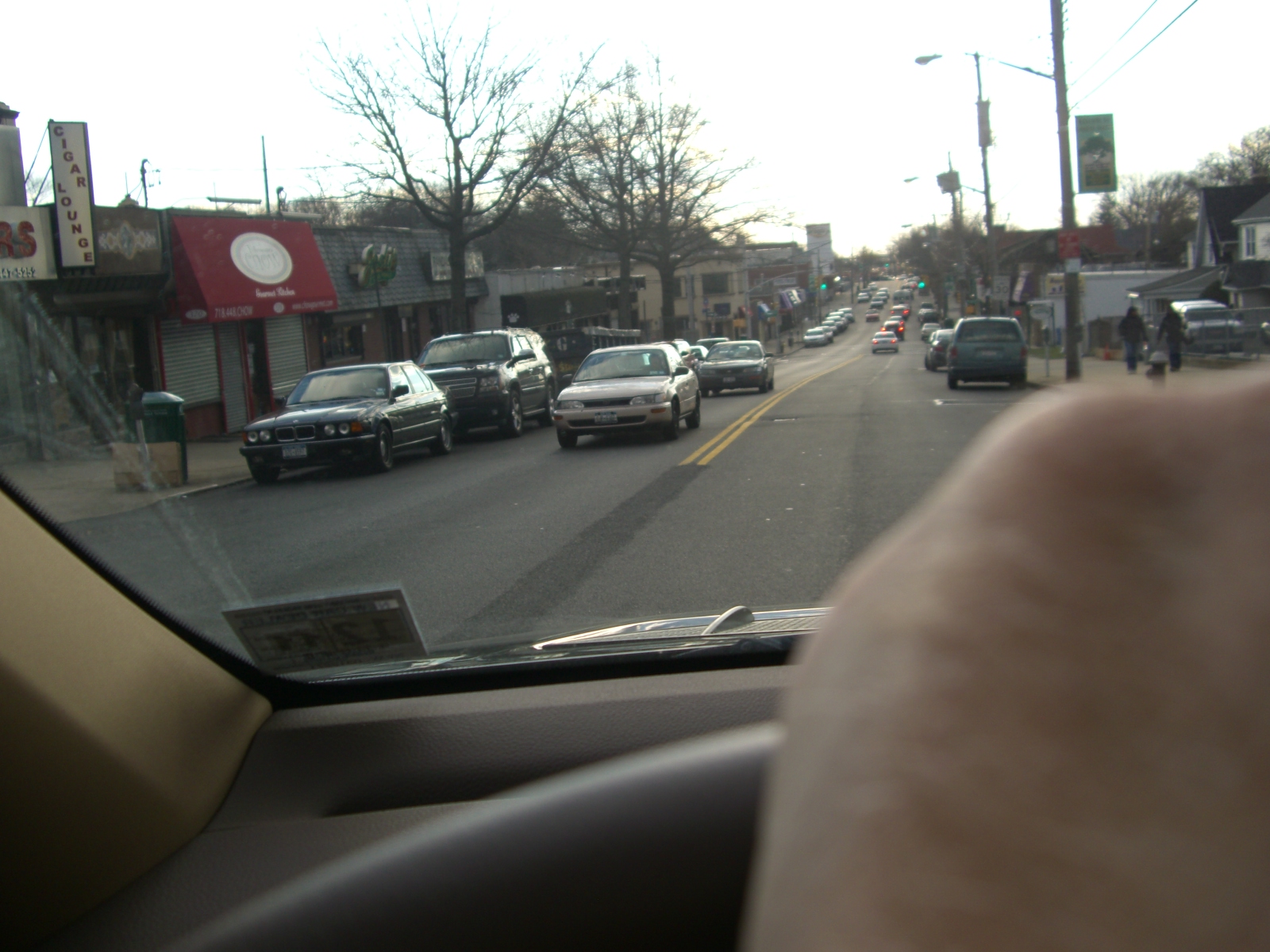This photograph captures a bustling downtown scene of a small town, likely from the mid-1990s, as suggested by the vintage body styles of the numerous vehicles scattered throughout the image. The street, lined with two lanes of traffic separated by a distinct yellow line, is flanked by various businesses on both sides, showcasing the town's commercial activity. Sparse trees, possibly indicating the early days of spring, are sporadically positioned along the sidewalks. The available on-street parking is entirely occupied, emphasizing the area's vibrant, busy atmosphere with numerous cars navigating and populating the scene.